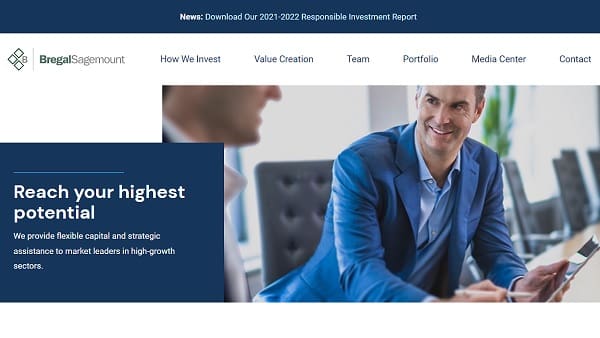The web page features a header with a prominent blue rectangular box that reads, "News: Download our 2021 to 2022 Responsible Investment Report." Below this, the header section displays the website's logo, consisting of three triangles and an '8' to the right of the triangles, followed by the text "Regal SageMount." 

A navigation menu is available offering options such as "How We Invest," "Value Creation," "Team," "Portfolio," "Media Center," and "Contact."

The main content area includes two sections. On the left, a blue box contains the inspiring message, "Reach your highest potential. We provide flexible capital and strategic assistance to market leaders in high-growth sectors," displayed in white text. To the right, there is an engaging photograph of two men. One man is partially visible in silhouette, and the other, dressed in a blue jacket and a blue-collared shirt, is smiling as they both look at a phone or an iPad. They are seated on black chairs around a brown table.